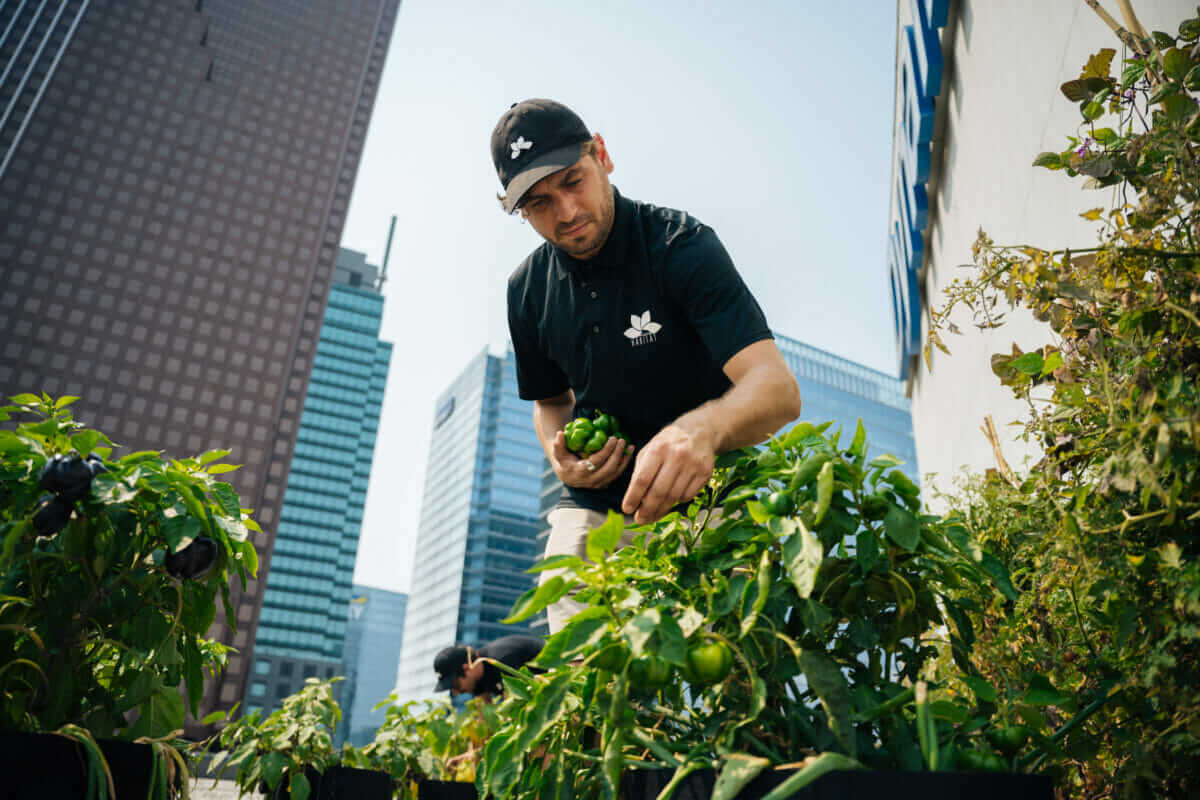In this rectangular outdoor image, wider than it is tall, we see a scene set against a backdrop of tall skyscrapers, including a prominent brown one, a bluish-silver one, and another on the right featuring indiscernible writing. Dominating the foreground, a man dressed in a black t-shirt and black hat, both adorned with an unreadable white flower-like logo, picks small green produce, possibly green tomatoes. Green plants span from the bottom to halfway up the right and left sides of the image. Another similarly dressed man, bent over and seemingly engaged in the same activity, appears in the background. The lush green plants and urban skyscrapers suggest a community garden or food co-op in a bustling downtown area, adding to the scene's vibrant juxtaposition of nature and city life.